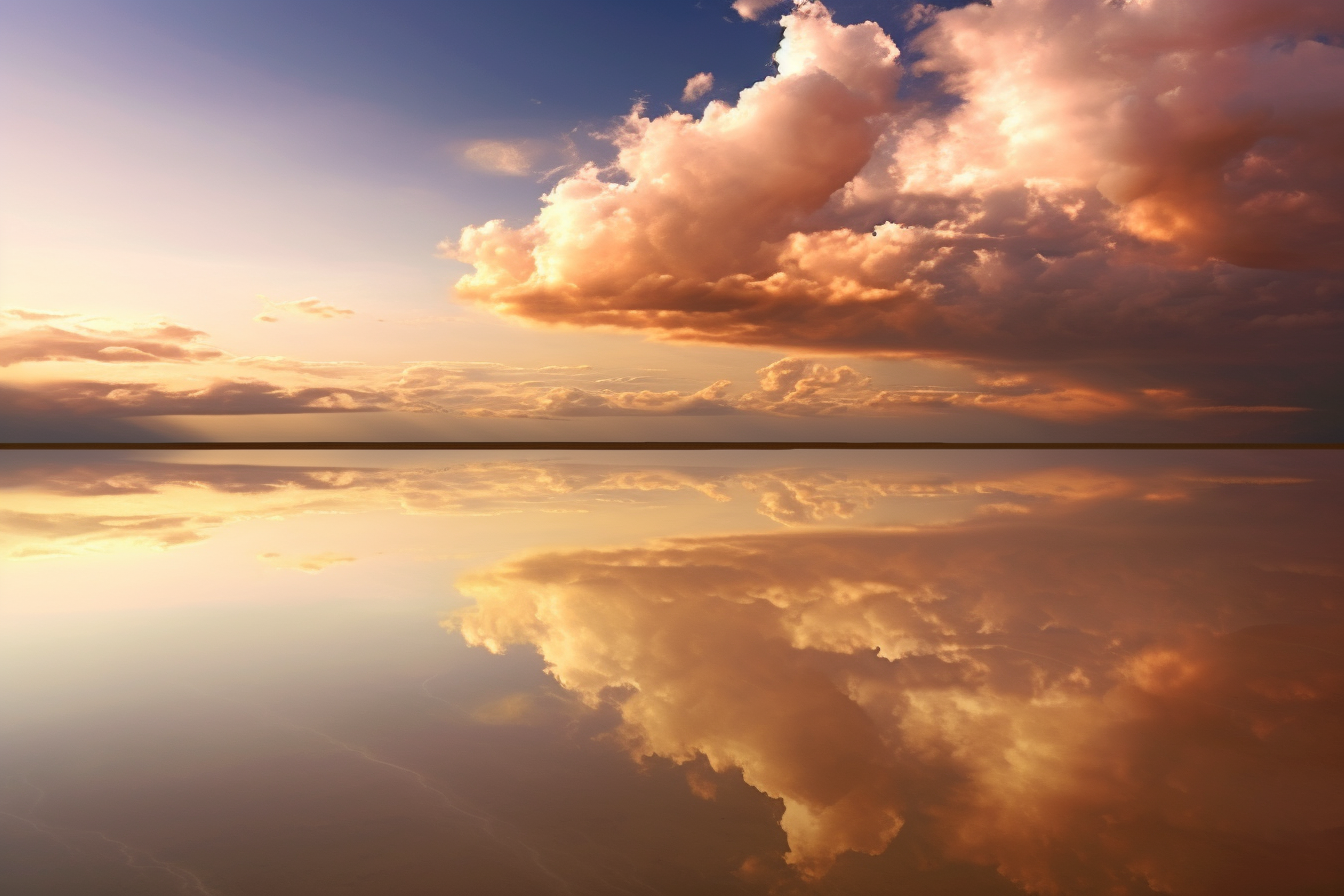This photograph captures a serene and symmetrical scene of a perfectly flat lake reflecting the sky above. The image is split horizontally by a thin, dark line representing the horizon where the water meets the sky. The top half of the photograph features a dynamic sky transitioning from a deep blue at the top to lighter shades as it approaches the horizon, with an array of clouds displaying a range of colors. On the right side, the clouds exhibit a pink-orange hue hinting at a sunrise or sunset just off-frame, while darker, storm-like clouds linger beneath them. The bottom half of the image is a mirror-like reflection of the sky, with the same cloudy formations and color transitions perfectly mirrored on the water’s surface. This symmetrical composition, with no humans or text, emphasizes the tranquil beauty of nature in this landscape shot.